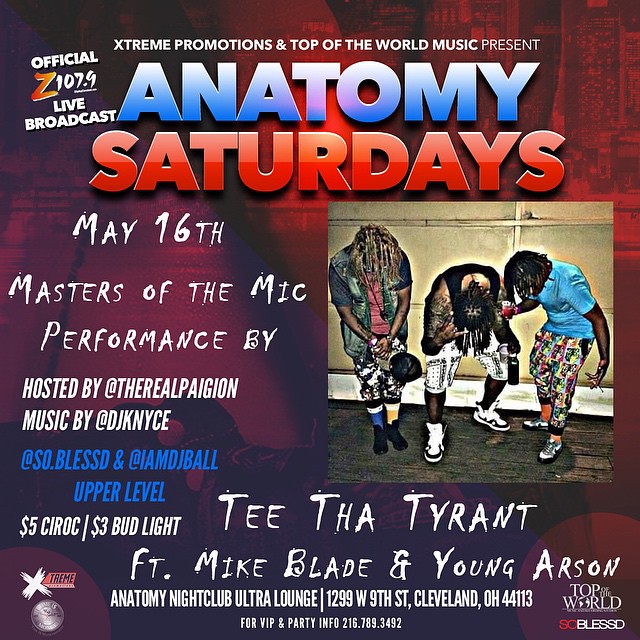The flyer promotes Club Anatomy’s "Anatomy Saturdays" hosted in Cleveland, Ohio. At the top, in white text, it reads "Extreme Promotions and Top of the World Music Presents," followed by the event title "Anatomy," depicted in bold blue uppercase letters that gradient to a lighter shade, and "Saturdays" in bold red uppercase letters. The left side features a smaller text, "Official Z107.9 Live Broadcast." Below this, the date "May 16th" appears in a scratch-out font alongside "Masters of the Mic Performance." Hosted by @TheRealPaigion and music by @DJKNICE, this section names T The Tyrant, Mike Blade, and Young Arson as performers.

Underneath, in blue text difficult to read against the darkened red background with black streaks, the flyer includes @Sodoblesto and @IMDJBALL. A promotional offer is listed in white uppercase letters: "$5 Ciroc / $3 Bud Light." At the very bottom, the location details read "Anatomy Nightclub Ultra Lounge / 1299 West 9th Street, Cleveland, Ohio 44113," with a contact number for VIP and party information. Logos for Top of the World and another possible logo are displayed at the bottom corners.

A significant visual on the flyer is a photo of three men—seemingly headbanging with dreadlocks, dressed in colorful shorts and sneakers—standing on a wooden floor against a beige wall, adding a dynamic element to the advertisement.